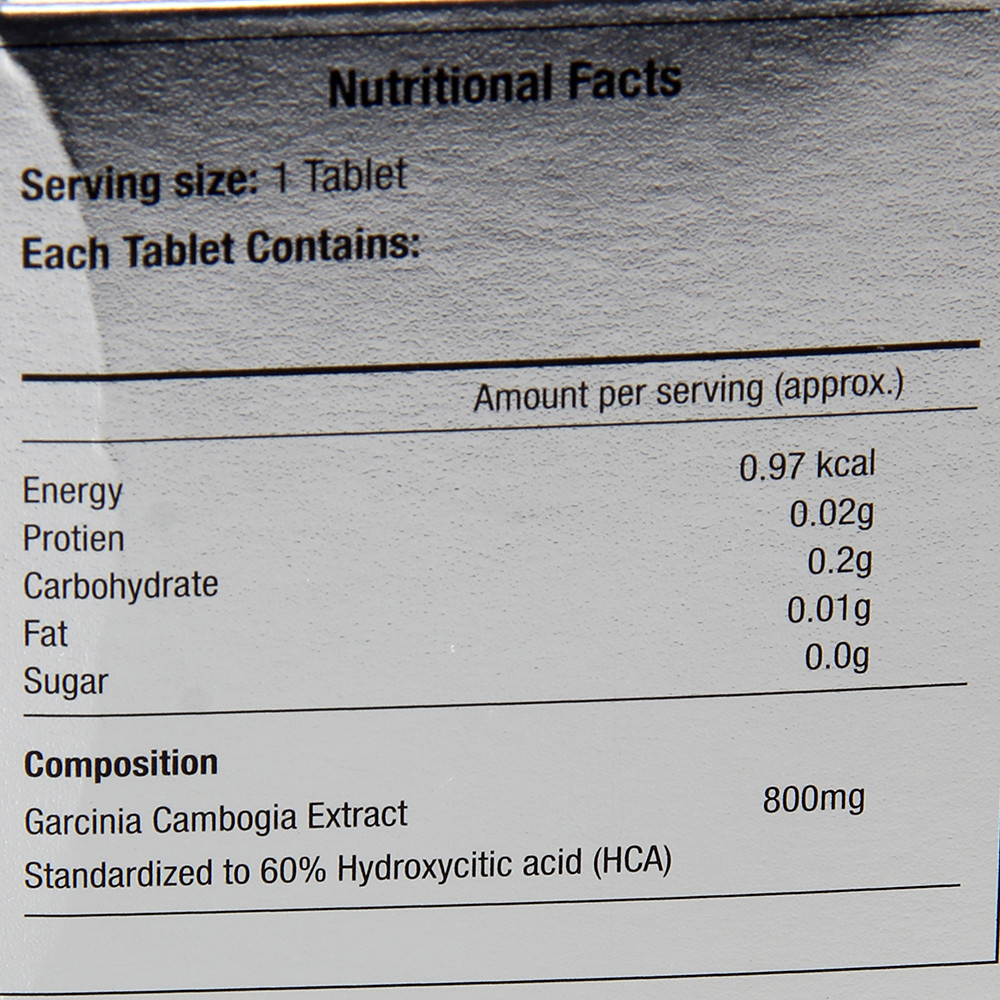This is a high-contrast black and white image of a nutritional facts label, presented in a square format on a white background. The text on the label is rendered in black for clear readability. At the top, the label prominently displays the heading "Nutritional Facts." Below this, it specifies the serving size as "One tablet" and continues with "Each tablet contains." Further down, it states "Amount per serving (Approx.)."

The nutritional information is organized into two columns. On the left column, from top to bottom, it lists:
1. Energy
2. Protein
3. Carbohydrate
4. Fat
5. Sugar
6. Composition

Beneath "Composition," it mentions the ingredient "Garcinia," with its spelling provided as "G-A-R-C-I-N-I-A." This detailed layout ensures that all pertinent nutritional information is easily accessible and legible.